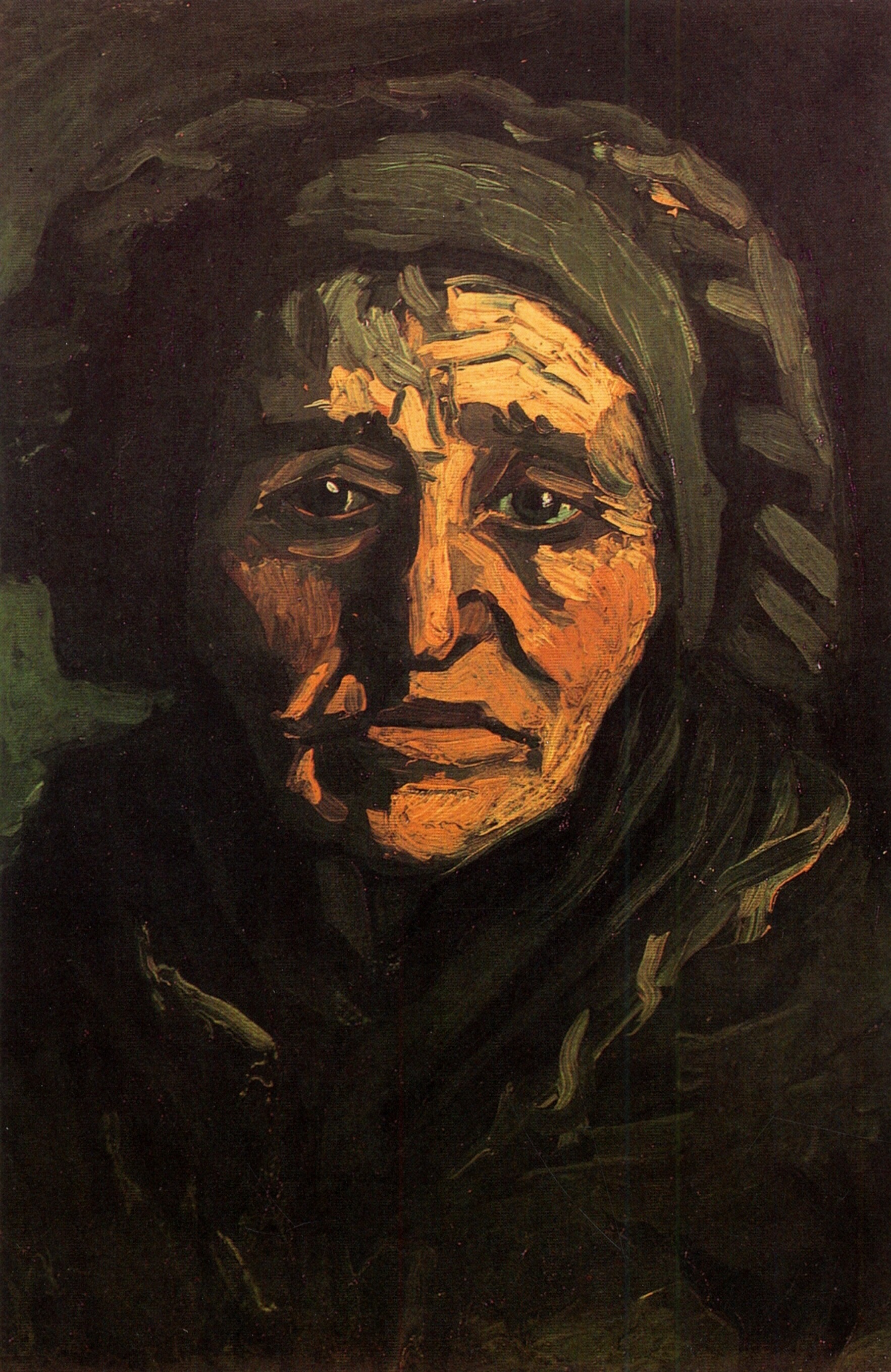Captured in this evocative painting is the poignant visage of an elderly woman, her deeply lined face rendered with skillful brushstrokes in shades of brown and orange, imbuing her skin with a somber, almost ethereal quality. Her gray hair peeks subtly from beneath a dark headdress that melds seamlessly into the similarly dark background, adding to the composition’s melancholic atmosphere. The woman's eyes are slanted and imbued with a haunting sadness, further emphasized by indented, worried brows that suggest a life of tribulation. Her attire, a black robe or outfit, is difficult to delineate against the shadowy backdrop, reinforcing the viewer's focus on her expressive, weary face. The style and attire hint at a period from the 18th or 19th century, giving the impression of a time long past, filled with untold stories and quiet despair.